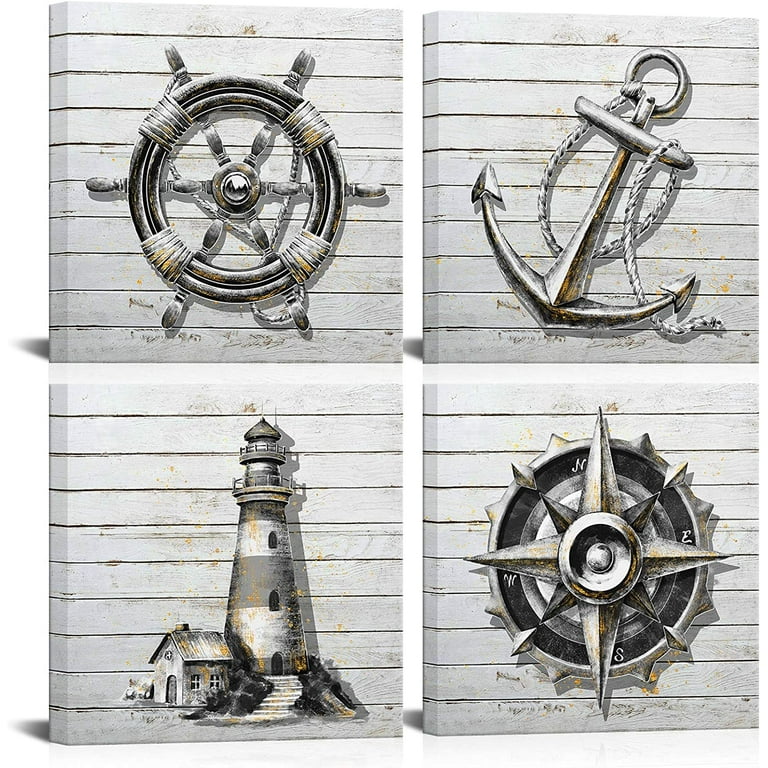The image comprises four distinct, unframed prints arranged in a 2x2 grid on a wooden-like material with a white background. Each print exhibits a maritime theme rendered in black and white. The top left print depicts a black ship’s steering wheel with white ropes intertwined, conveying the sense of nautical navigation. Adjacent to it, the top right print features a tipped anchor with arrowheads at both ends, symbolizing stability and direction. The bottom left print showcases a detailed lighthouse with an attached tiny house, capturing the essence of coastal life. Finally, the bottom right print presents a compass with a star-like design, emphasizing exploration and guidance. The prints collectively evoke a coastal and seafaring atmosphere, emphasizing a cohesive water-themed aesthetic with artistic, animated touches.